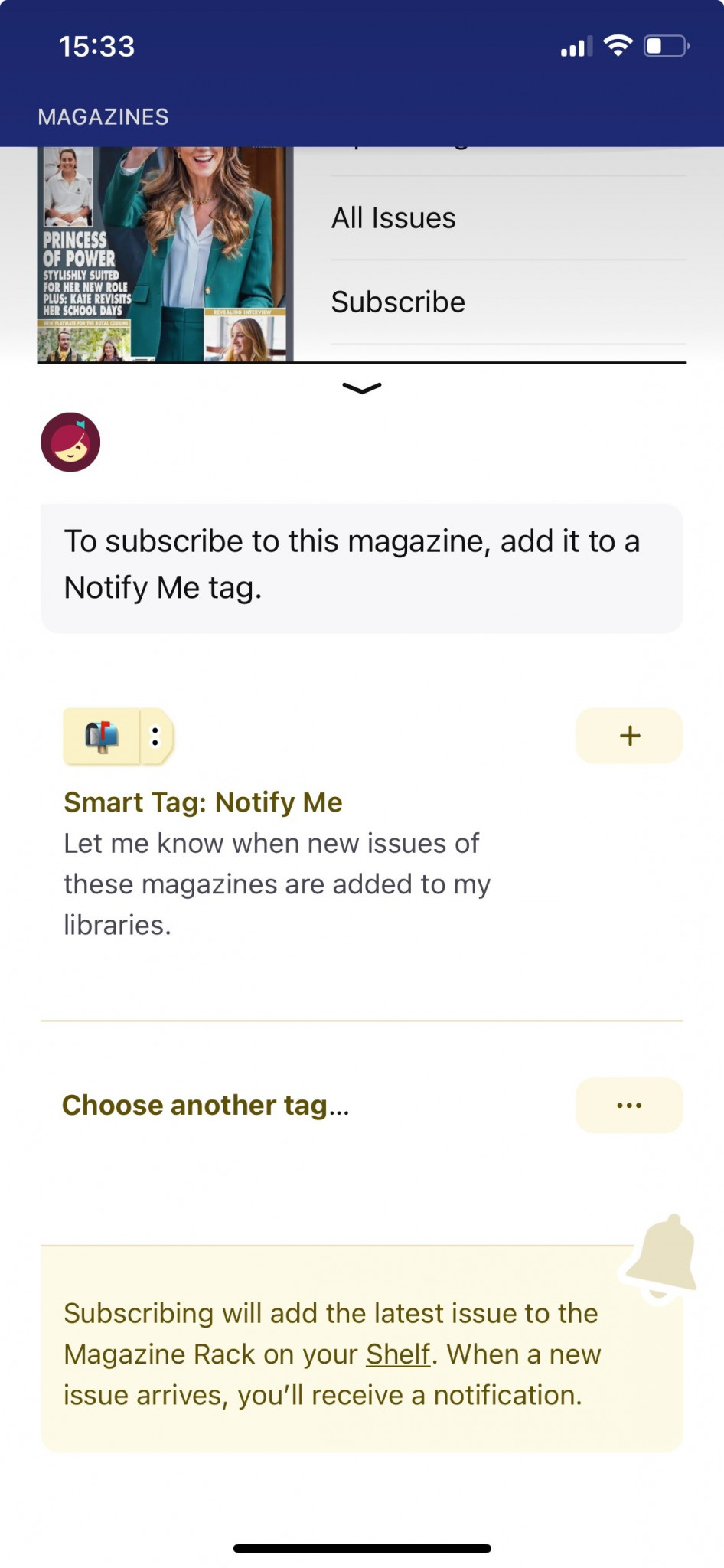Category: Websites

In the image, a smartphone screen displays a website interface related to magazine subscriptions. The time on the phone is 15:33, as indicated on the top right corner of the screen. The device is connected to Wi-Fi and shows a battery level of approximately 25%. 

At the top of the screen, within a blue bar, the word "Magazines" is prominently displayed in white letters. Just below this, there is a partial magazine cover featuring a woman dressed in a teal suit and white shirt, though her face is cropped from the nose down. Accompanying the image, in gray text, are the words "All issues are subscribed."

Further down, the website provides users with the option to subscribe to the featured magazine. It prompts users to "Add it to a Notify Me tag" to receive updates. Next to this instruction, there is a small mailbox icon accompanied by the text "Smart Tag. Notify Me. Let me know when new issues of these magazines are added to my libraries," alongside a plus sign for adding the tag.

The interface also provides an option to "Choose another tag," represented by three horizontal dots that likely open additional settings or options. A helpful note explains that "Subscribing will add the latest issue to the magazine rack on your shelf," and when a new issue is available, "You'll receive a notification," shown with a notification bell icon.

The magazine cover at the top also includes a small image of another person dressed in white, but the details are too small to discern their gender. Overall, the website offers an intuitive option for users to subscribe to their favorite magazines and receive timely updates whenever new issues are released.